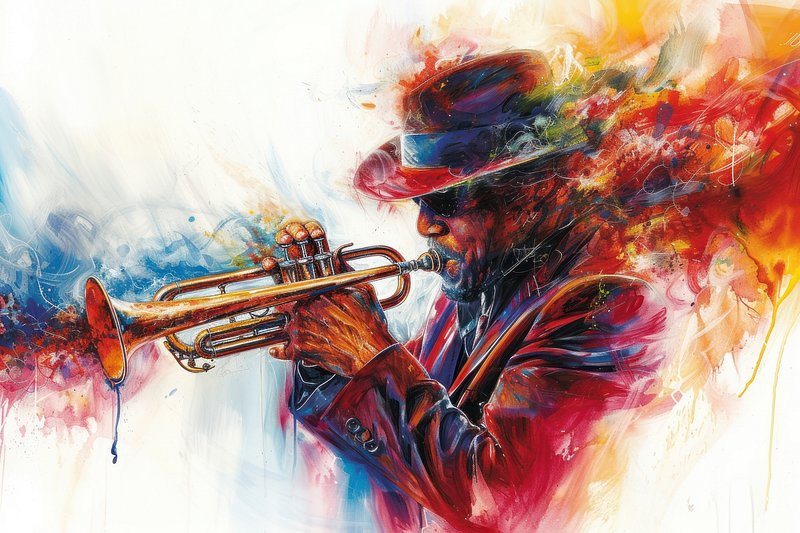The image is a vivid, colorful painting of an African American man playing a trumpet, set against a predominantly white background. The man is dressed sharply in a suit jacket, with a hat featuring a stripe band just below the crown, and he sports sunglasses and a neatly groomed beard with a mustache. His right hand expertly presses the valves of the trumpet, while his left hand supports it. The instrument features blue colors dripping from its bell, and it expels vibrant wisps of pink, purple, blue, yellow, red, magenta, orange, gold, and silver, blending in tie-dye like fashion. These bursts of colors are fluid and dynamic, resembling watercolors or paint strokes, adding a sense of rhythm and movement to the piece. The bright hues and energetic composition evoke the soulful essence of a blues trumpet player.